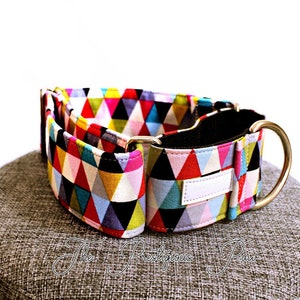The image depicts a padded brown stool with a circular pattern, featuring light brown cursive text that is difficult to read due to blending with the fabric. Resting on the stool is a wide, heavy-duty dog collar adorned with an eclectic array of colorful triangles, including shades of red, pink, light blue, black, purple, and teal. These triangles are arranged in alternating directions across three rows, bordered by thin lines of stitching. The collar also has a brass loop affixed to the front, which appears to be reinforced by double-layer stitching. The stool itself is placed against a vibrant, pure white background, enhancing the contrast and visual appeal of the scene.